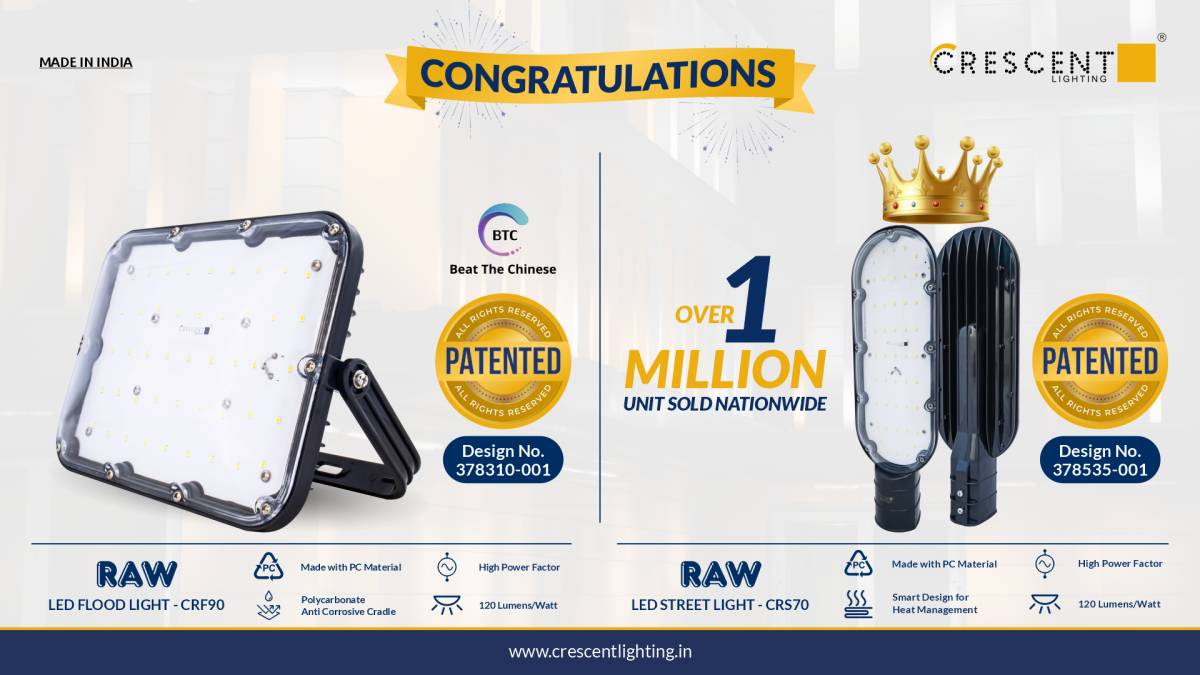This advertisement for Crescent Lighting features a white background adorned with a celebratory theme. Centered at the top is a yellow ribbon with the blue inscription "Congratulations," enhanced by fireworks in the background. To the right of the ribbon is the Crescent Lighting logo, which includes a yellow square box with a crescent shape above the 'C', and a small 'R' in a circle indicating a registered trademark.

On the left side of the image, a RAW LED floodlight is displayed, accompanied by its serial number CRF90 and a gold patented stamp with the design number 38730001. An icon indicating "Made with PC material" (polycarbonate) and a symbol denoting "anti-corrosive cradle" can also be found near the floodlight. On the right side, there is a RAW LED street light, also bearing a serial number and the gold patented stamp. This light has a crown icon above it and a caption stating "over 1 million units sold nationwide." Additional icons indicate high power factor and 120 lumens per watt efficiency for both products. 

At the bottom of the advertisement is a blue strip featuring the URL: www.crescentlighting.in, guiding viewers to the company's website for more information.